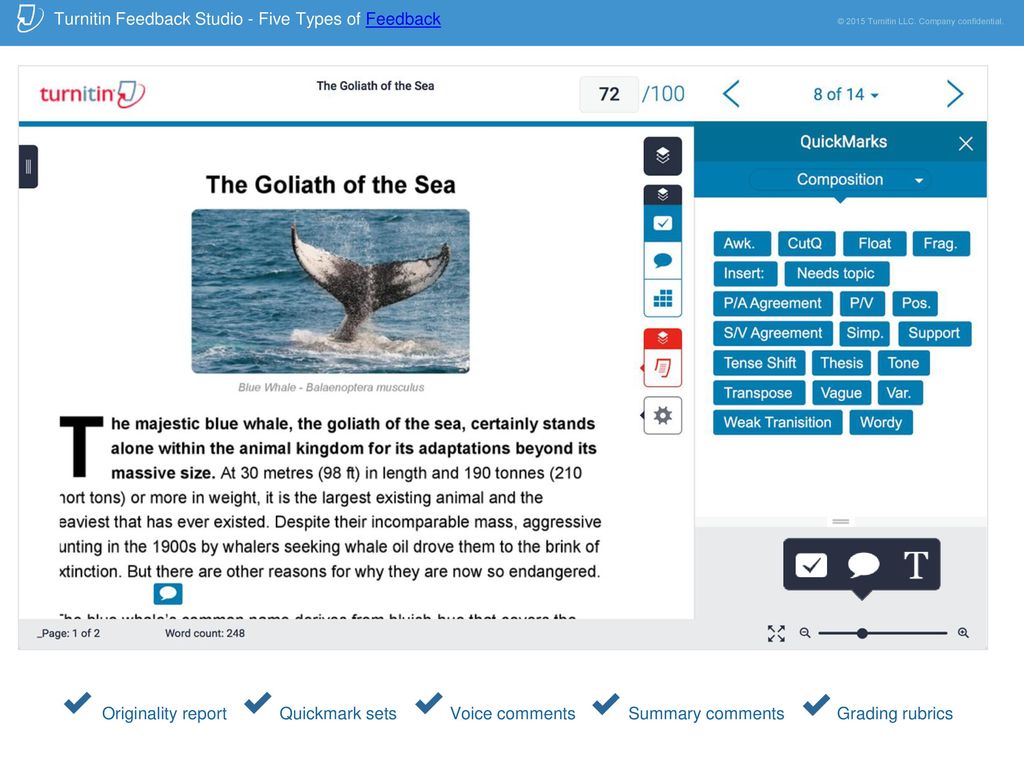The image features a webpage from TURNITIN Feedback Studio entitled "Five Types of Feedback," characterized by a prominent blue band across the top. On the left side of the blue band, the text "TURNITIN Feedback Studio" is displayed. To the right of the band, it reads "Copyright 2015, Turnitin LLC Company Confidential."

The main content of the page begins with the title "Turnitin: The Goliath of the Sea," accompanied by a detailed description of the blue whale, often referred to as the "Goliath of the Sea." The text explains the enormity of the blue whale, highlighting its massive size of up to 30 meters (98 feet) in length and a weight ranging from 190 tons to over 210 tons, making it the largest and heaviest animal to ever exist. Despite their massive size, aggressive hunting for whale oil in the 1900s brought blue whales to the brink of extinction, although other factors also contribute to their endangered status. 

The left margin of the document appears slightly cut off, omitting the initial letters from words such as "heaviest," "hunting," and "extinction," showing them as "eaviest," "unting," and "xtinction" respectively. This document is labeled as "Page 1 of 2" and has a word count of 248.